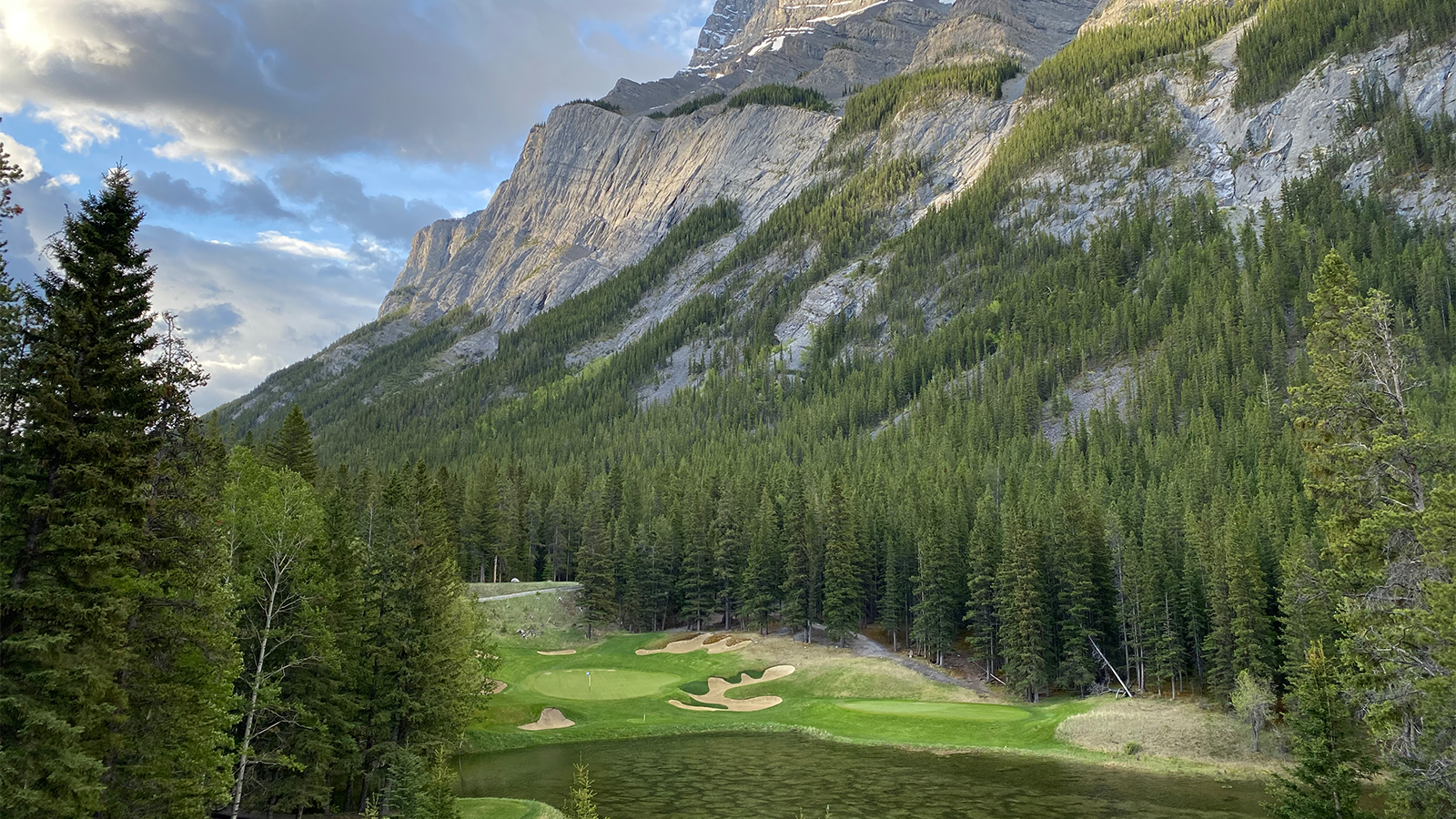The image depicts a picturesque mountain forest landscape dominated by a towering, rocky mountain in the background. The sky is light blue with patches of grayish-blue and white clouds, through which sunlight is streaming. The lush, green forest ascends the mountain, primarily composed of tall pine trees, creating a densely wooded scene. On the left-hand side, tall pine trees stand prominently with more trees receding into the background.

In the center and towards the bottom of the image, there is a vibrant green golf course nestled within a large valley. This golf course features several sand traps and a small, dark green lake, which may be reflecting the surrounding forest. The course is flat and well-maintained, with some patches of lighter green grass. There appears to be a flag on one of the golf pits, and at the edge of the golf course, there is a structure resembling a road or wall.

The overall ambiance suggests a serene and natural setting, possibly captured in early spring or later in the day. The intricate details of the landscape, from the verdant forest to the majestic mountain, paint a vivid picture of this captivating and tranquil environment.